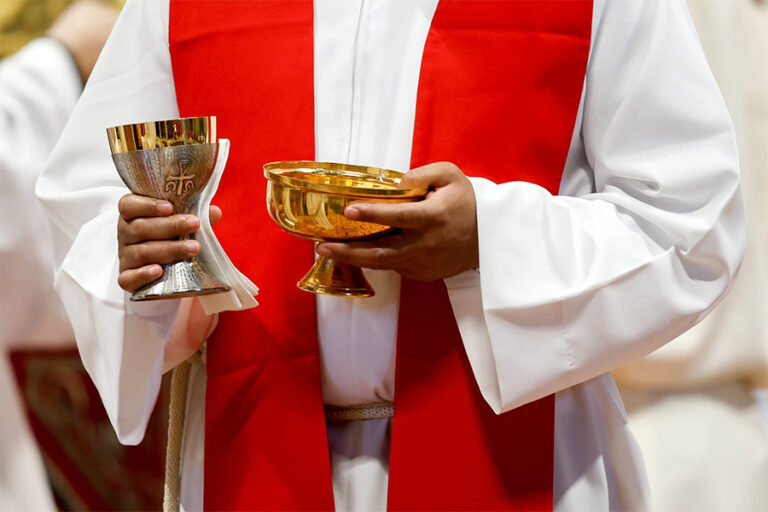In this photograph taken during a religious ceremony inside a church, a Catholic priest, whose face is cropped out of the image, is depicted holding two chalices. The priest is dressed in a traditional white robe adorned with a wide-sleeved design and a red sash that drapes over his shoulders. Additionally, a tan-colored tassel rope further embellishes his outfit. With his left hand, the priest holds a short, shiny golden chalice, likely used for the bread sacrament of communion. In his right hand, he holds a taller, ornate chalice featuring a golden upper section with crosses and symbols, tapering into a silvery lower part. This chalice is presumably used for wine during the communion. The right-hand chalice includes intricate icons, possibly an Ankh symbol flanked by Omega symbols, suggesting a deeper cultural or symbolic significance. Other clergy members, dressed in similar white robes, are visible but slightly out of focus in the background, emphasizing the ceremonial context. A light source from overhead illuminates the scene, confirming the indoor setting of the church and casting reflections that vaguely indicate a carpeted floor.